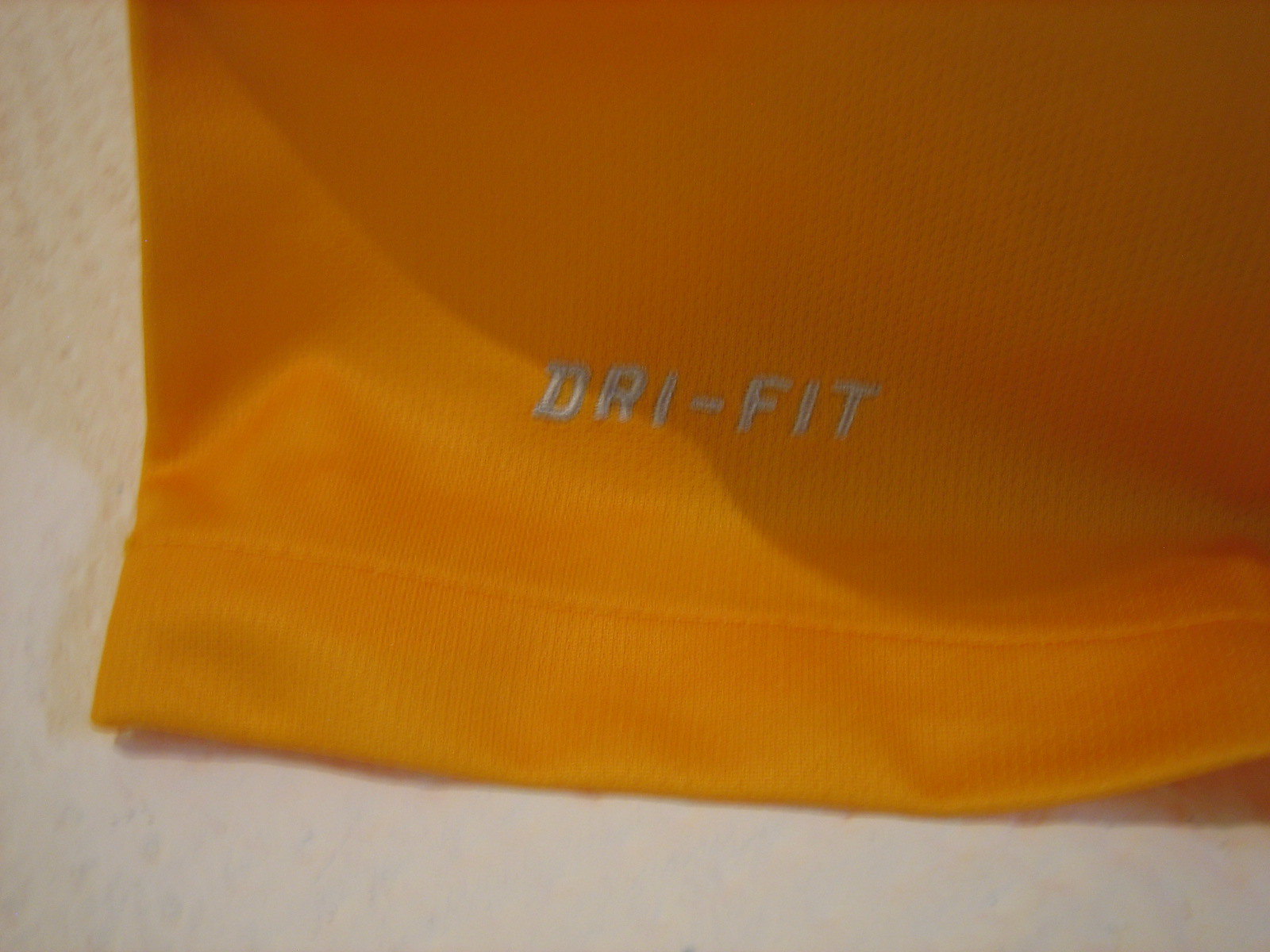In this image, we see a detailed close-up of the bottom corner of an orange t-shirt, which is laid out on a white, textured cloth surface. The t-shirt casts a discernible shadow on the cloth, emphasizing the fabric's presence. The orange hue of the t-shirt is vivid, and there is precise orange stitching about an inch above the hem, which runs horizontally across the garment. Above the hem, approximately three to four inches of the t-shirt’s woven fabric are visible, revealing its intricate fibers. Notably, the lower part of the t-shirt displays the word "DRI-FIT" stitched in white. The lighting in the image creates a gradient of shadows, with the top right corner appearing darker compared to the lighter bottom left corner.